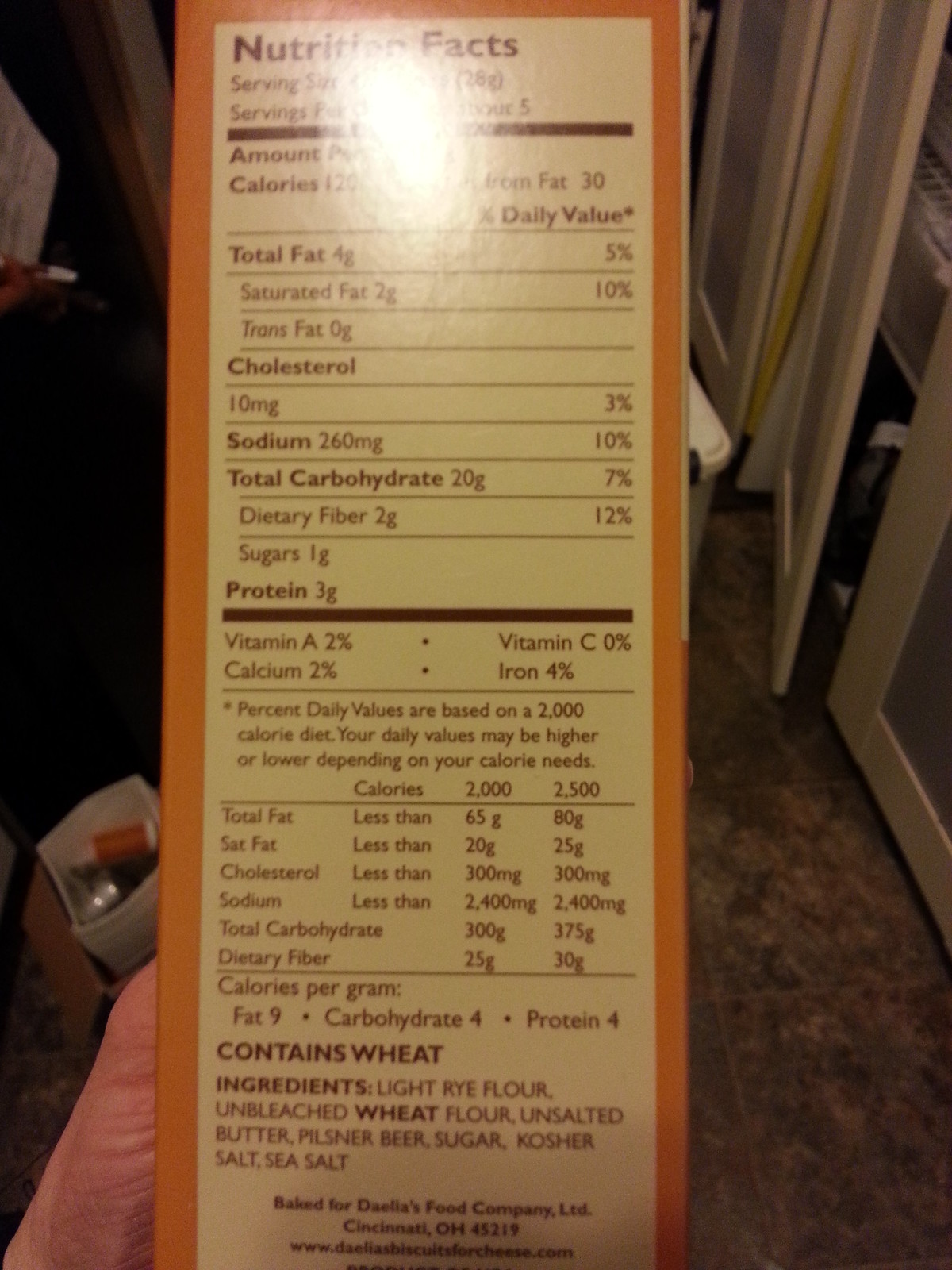This photograph captures the side of a rectangular packaging, presumably for crackers, evident from its design and typical labeling. The top of the packaging features the phrase "Nutritional Facts," though a bright reflection obscures the detailed information beneath. Dominating the center and running vertically down the middle is a list of the product’s ingredients, making them the focal point of the image. Highlighted ingredients include wheat, light rye flour, unbleached wheat flour, unsalted butter, pilsner beer, sugar, kosher salt, and sea salt. The box itself is a striking combination of orange, white, and black colors. In the background, a carpeted floor is visible, along with partially seen doors, some fabric, and an indistinct box of unidentified items, contributing to a homey, lived-in ambiance.